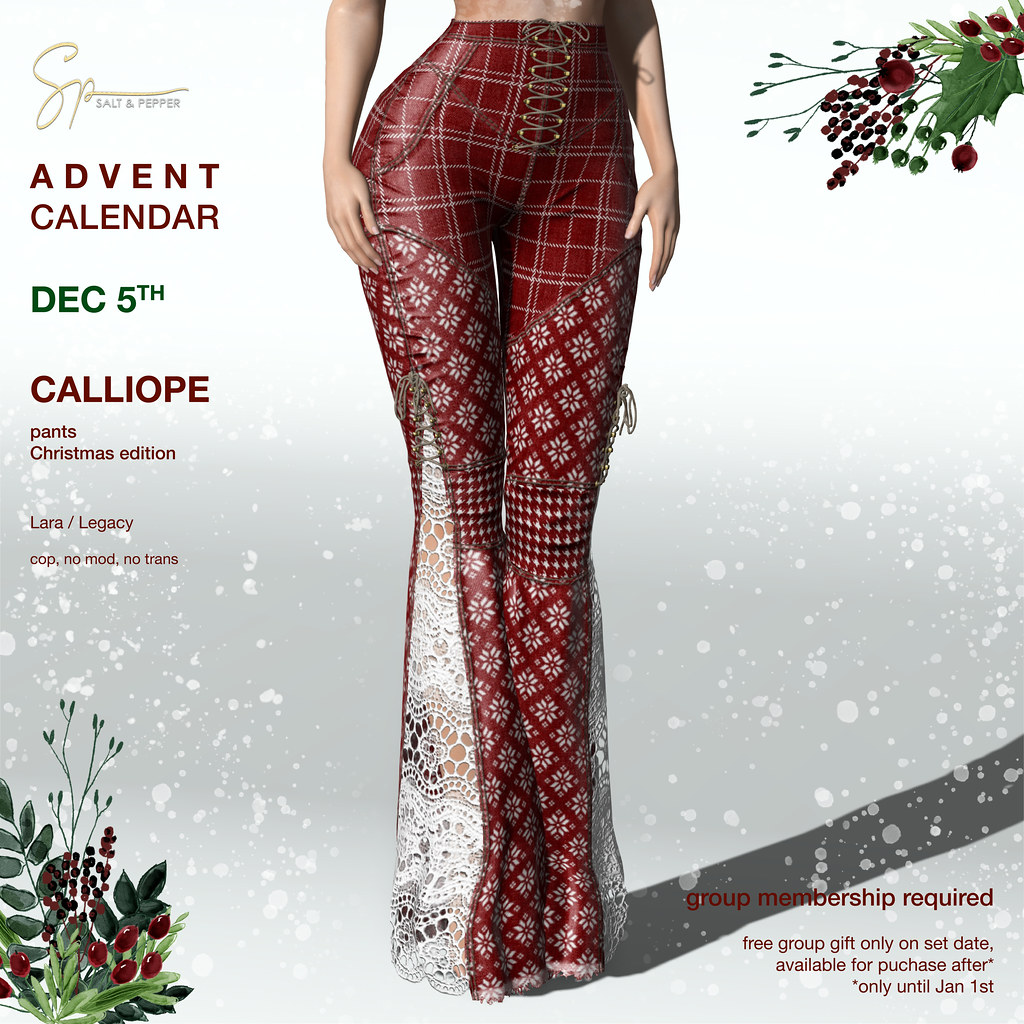The image is a vibrant advertisement, likely computer-generated or meticulously illustrated, showcasing the bottom half of a woman wearing festive red leggings. These luxurious leggings, made from a material resembling leather, are adorned with intricate snowflake patterns and delicate lace running along the sides. A variety of interwoven lines and patterns, including gray intersecting lines and houndstooth near the knees, add a rich texture to the design. Decorative string ties cinch the leggings at the waist, completing the festive look.

On the left side of the image, in elegant gold cursive, it reads "SP" followed by "Salt and Pepper". Below this, "Advent Calendar" is prominently displayed in red font, with "December 5th" in green. The leggings are identified as the "Calliope Pants Christmas Edition", suitable for the Lara and Legacy bodies, with a note specifying "Cop No Mod No Trans." The bottom right corner mentions that these leggings are a "group membership required, free group gift" only available on the set date, with purchases allowed until January 1st. The corners of the image are adorned with drawn sprigs of holly and red berries, adding an additional touch of holiday spirit.